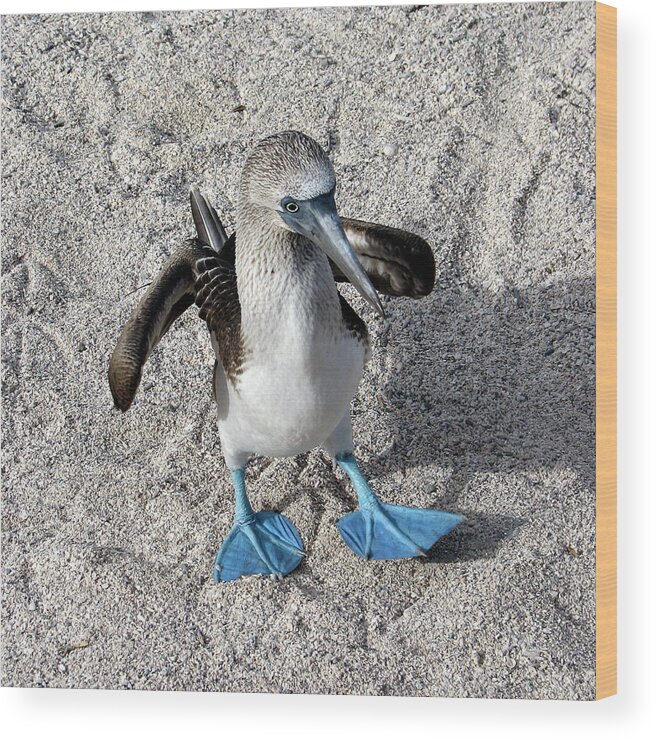This is a color photograph taken from a high vantage point, depicting a unique seabird standing on a gritty, gray sand surface. The seabird has a distinctive appearance with a white breast and a black and white head and neck. Its long, pointy bill is a dark gray shade. The bird's eyes are striking, featuring large black pupils surrounded by silver. Its wings, slightly extended to either side, are gray with darker feather tips, while its tail feathers are black with some white flecks visible. A noteworthy feature is its bright baby blue, webbed feet, which stand out starkly against its body. The seabird casts a shadow to the right on the sand, where footprints of similar birds are also visible. The entire image has the quality of being affixed to a light wood frame or canvas, enhancing its decorative appeal.